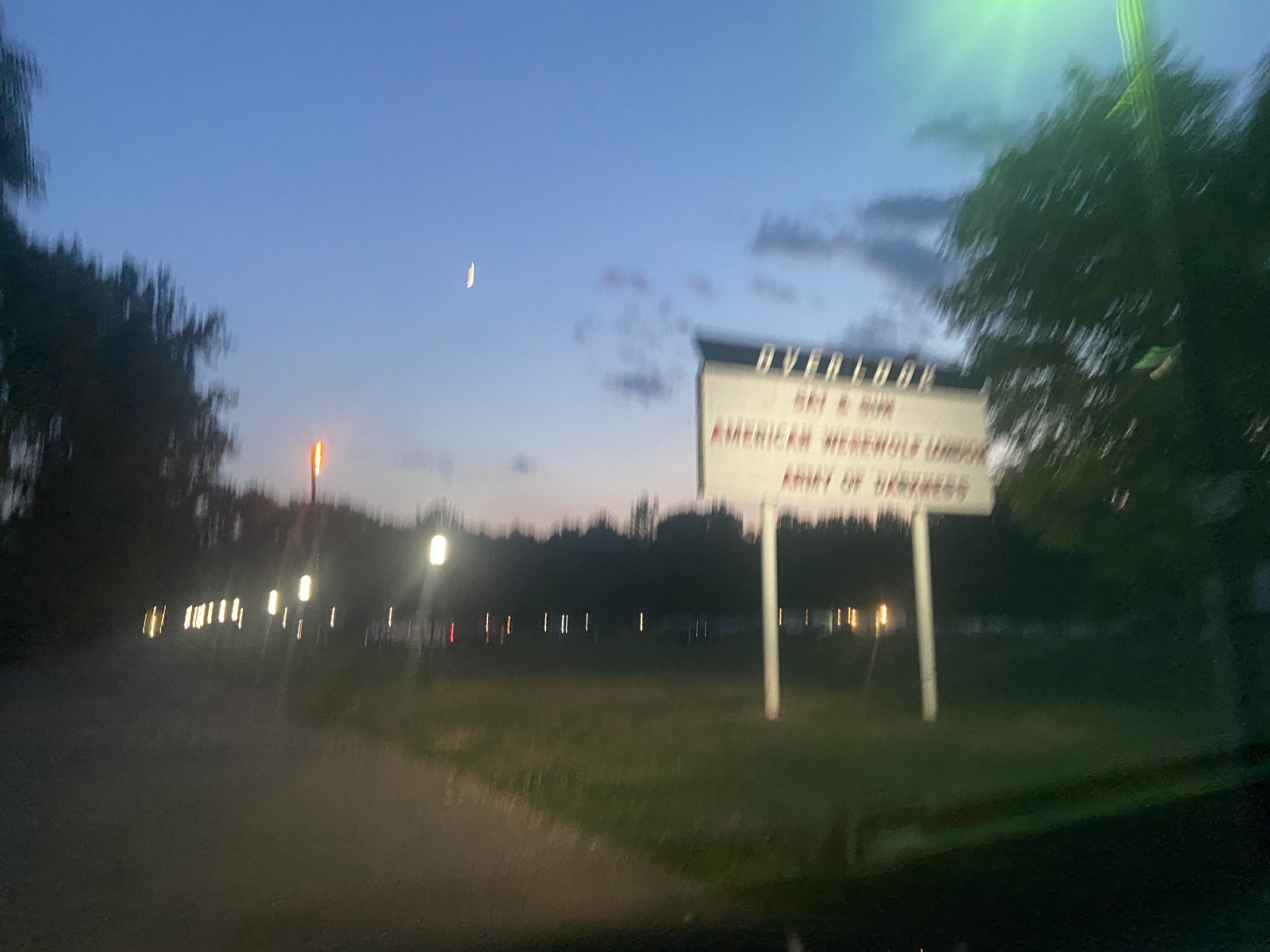A blurry color photograph, presumably taken at dusk, depicts an outdoor scene characterized by a tranquil yet eerie atmosphere. On the left side of the image, a dark, unlit road stretches into the distance, bordered by trees whose branches meld into the shadowy surroundings. To the right, a grassy area extends, populated sporadically with trees that cast long, dim shadows in the fading light. The sky transitions from a deep, dark blue at the top to a lighter hue nearer the horizon, suggesting the end of twilight.

In the background, several faint lights illuminate the scene, their sources unclear but contributing to a mysterious ambiance. Among the trees in the grassy area stands a white sign that reads "Overlook." The text beneath this heading is too blurry to decipher fully, but phrases such as "American Werewolf," "London," and "Army of Darkness" are distinguishable, hinting at a possible reference to cinematic themes, perhaps indicating the location is a drive-in theater.

No people, animals, or vehicles are present in the photograph, giving it a desolate and almost haunting feel.